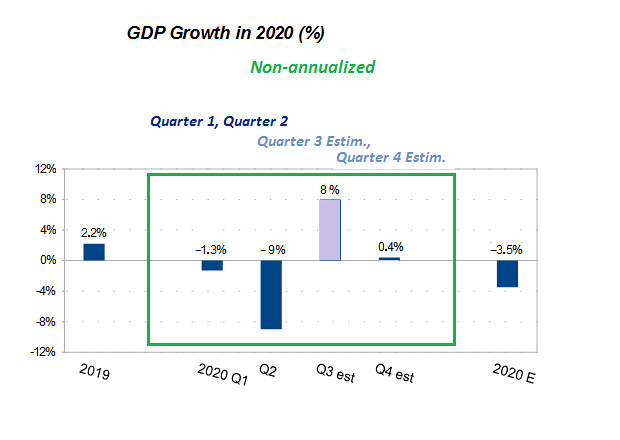The image is a detailed bar graph depicting GDP growth percentages in 2020, focusing on non-annualized quarterly data. The chart's title is "GDP Growth in 2020 (Percentage)" with "Non-Annualized" right below it. The quarters are labeled sequentially from Q1, Q2, Q3 Estimate, and Q4 Estimate. The y-axis, marked on the left, ranges from -12% to 12% in increments of 4%, with labels at -12%, -8%, -4%, 0%, 4%, 8%, and 12%. The x-axis starts from 2019 and spans through 2020 Q1, Q2, Q3 Estimate, Q4 Estimate, ending with 2020 E.

Bars are color-coded: gray bars indicate positive growth, and dark blue bars indicate negative growth. Specific data points include:
- 2019: 2.2% (positive growth, gray bar)
- 2020 Q1: -1.3% (negative growth, dark blue bar)
- 2020 Q2: -9% (negative growth, dark blue bar)
- 2020 Q3 Estimate: 8% (positive growth, gray bar)
- 2020 Q4 Estimate: 0.4% (positive growth, gray bar)
- 2020 E: -3.5% (negative growth, dark blue bar)

Two green horizontal lines emphasize thresholds at the top and bottom of the graph. The overall layout uses a white background and light gray axes for clarity, with percentage values on the y-axis and time periods (quarterly estimates) on the x-axis.